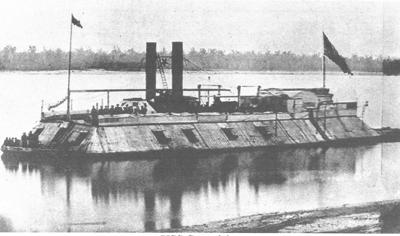This grainy, black and white vintage photo, likely from the early 1900s, depicts an old, industrial steel-plated ship, possibly of military origin, situated in a body of water. The ship, which has a trapezoidal shape with railings, is captured prominently in the center of the frame. Two flags are visible: a larger flag at the back (right side of the photo) and a smaller one at the front (left side of the photo). The vessel features distinct masts or pillars, and there are numerous ladders and what might be windows or cannon ports along its side. The ship's surface is populated by small, barely discernible figures, presumably crew members, who are scattered across its deck. The faint outline of trees can be seen in the background on the opposite bank, completing the historic, serene scene with the ship’s reflection mirrored in the water below.